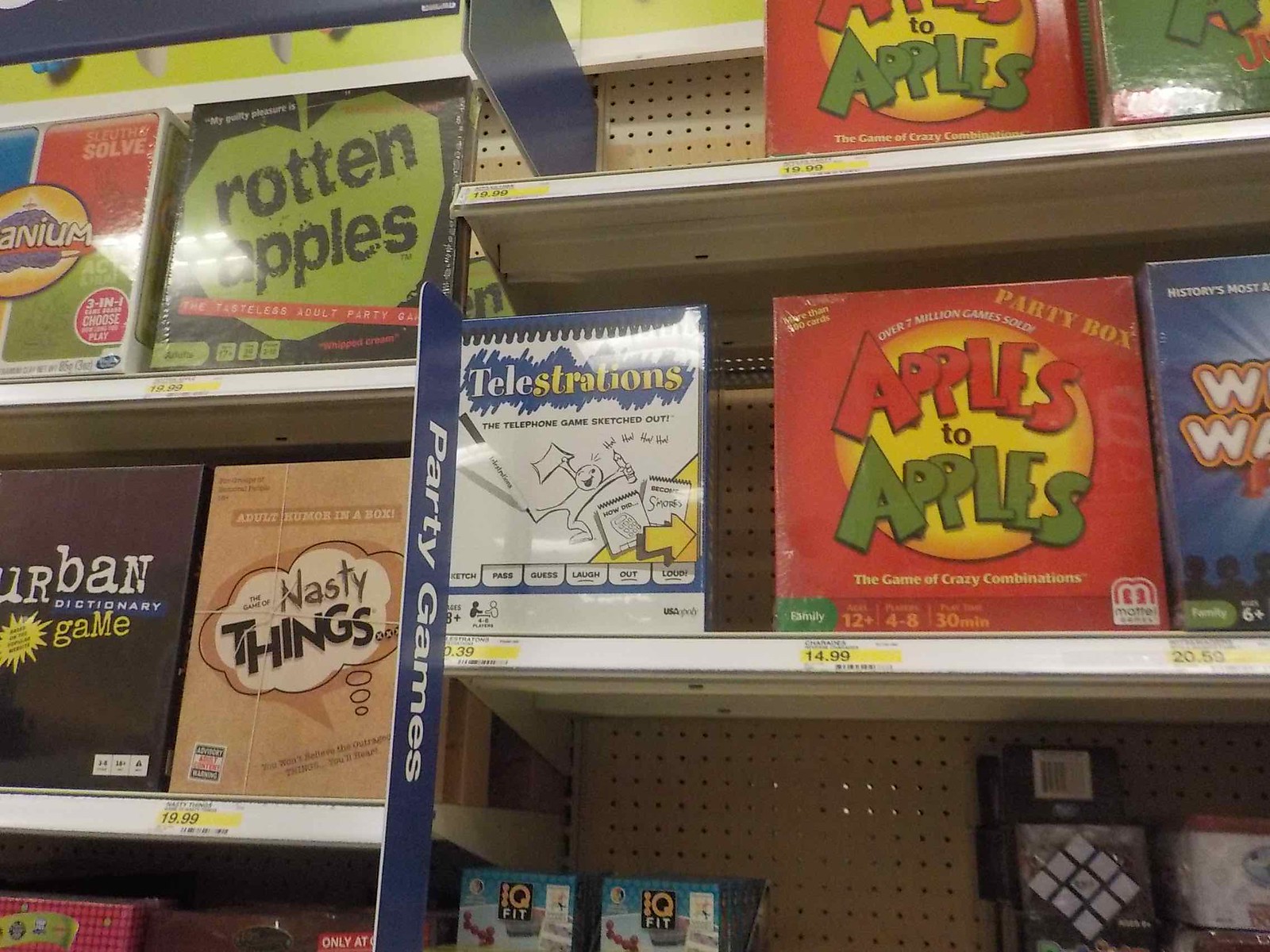The photograph captures a store shelf filled with board games, neatly arranged. At the top right, a prominent red box labeled "Apples to Apples" is priced at $19.99. Directly below it, a similar game titled "Apple to Apple" features the phrase "Party Box" on the top right corner and "The Game of Crazy Combinations" at the bottom, costing $14.99. Other visible games include "Cranium," "Rotten Apples," "Urban Dictionary Game," "The Game of Nasty Things," and "Telestrations," a white, blue, and yellow boxed game priced at $10.39. Another game with a blue box featuring "W's" is priced at $20.59. The shelves are beige and perforated, with yellow price tags marking each item's cost. The image also hints at a lower shelf partly visible, displaying two boxes labeled "QFIT."